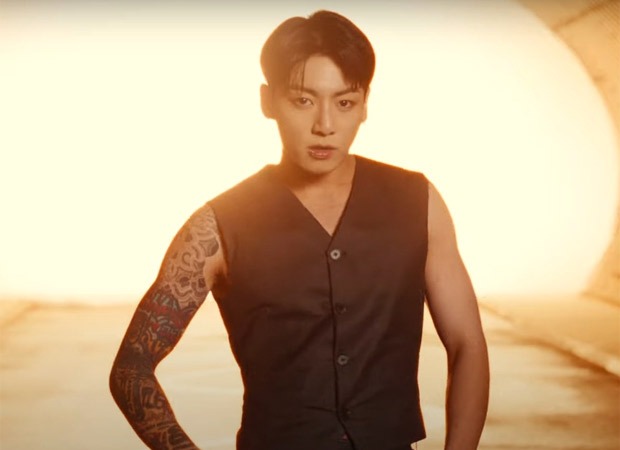The image features a young Asian man in his 20s, standing and looking directly at the camera with a serious expression. He has short, straight brown hair parted in the middle, reaching his eyebrows. The man is wearing a black vest with a V-neck and multiple buttons, which is unbuttoned down to the bottom, revealing that he has no shirt underneath. His right arm is adorned with a full sleeve of tattoos, which are predominantly black on his upper shoulder and gradually include red and blue hues as they extend down to his forearm, disappearing out of the frame.

The man stands with his right hand resting on his hip and his left arm relaxed at his side. The background behind him is very bright, mostly white with subtle yellow tones, particularly on the right side and towards the lower part of the image. The surroundings give an impression of a tunnel or a similarly illuminated space. The background is intentionally blurred, emphasizing the man's presence in the photo.